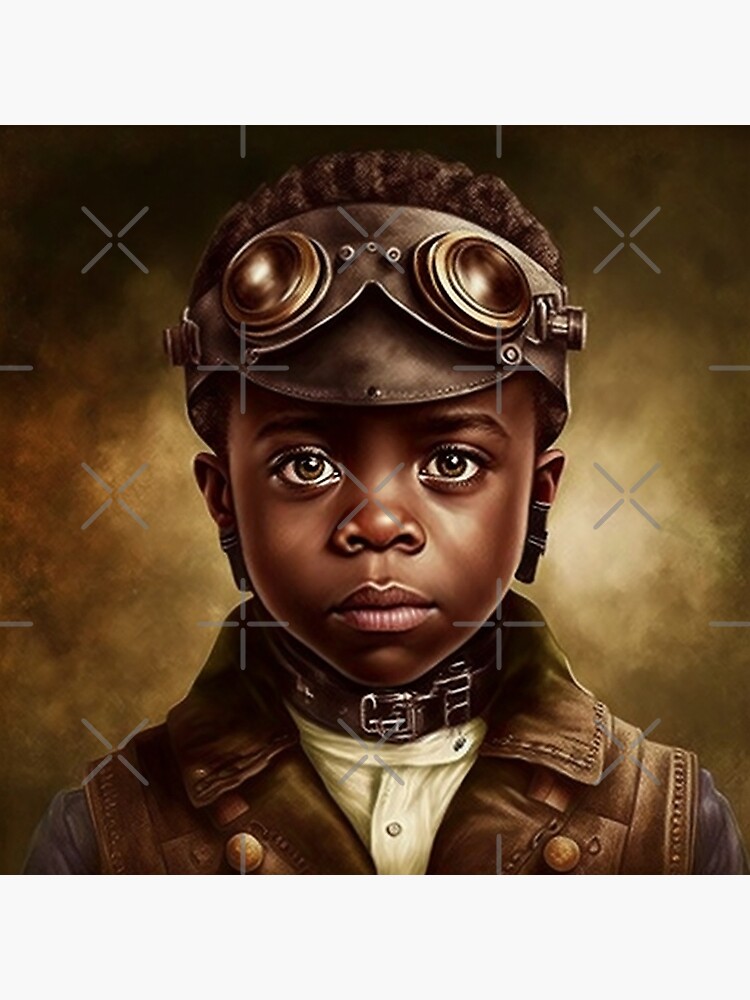The image is a detailed artwork of a young African-American boy with short, black curly hair and light brown eyes, wearing an aviator outfit. He dons a brown leather aviator jacket with a beige button-up shirt underneath. The jacket is adorned with brass buttons and chains, and he has an aviator cap that covers his ears, complete with goggles resting on his forehead. The goggle straps are black, with circular lenses. Around his neck, he sports a belt-like necklace with a silver buckle. The boy’s expression is noticeably sullen, conveying an unexpected sense of sadness. The background is a light brown and white blend, with white X's and pluses interspersed, adding a distinct texture to the golden-brown backdrop.